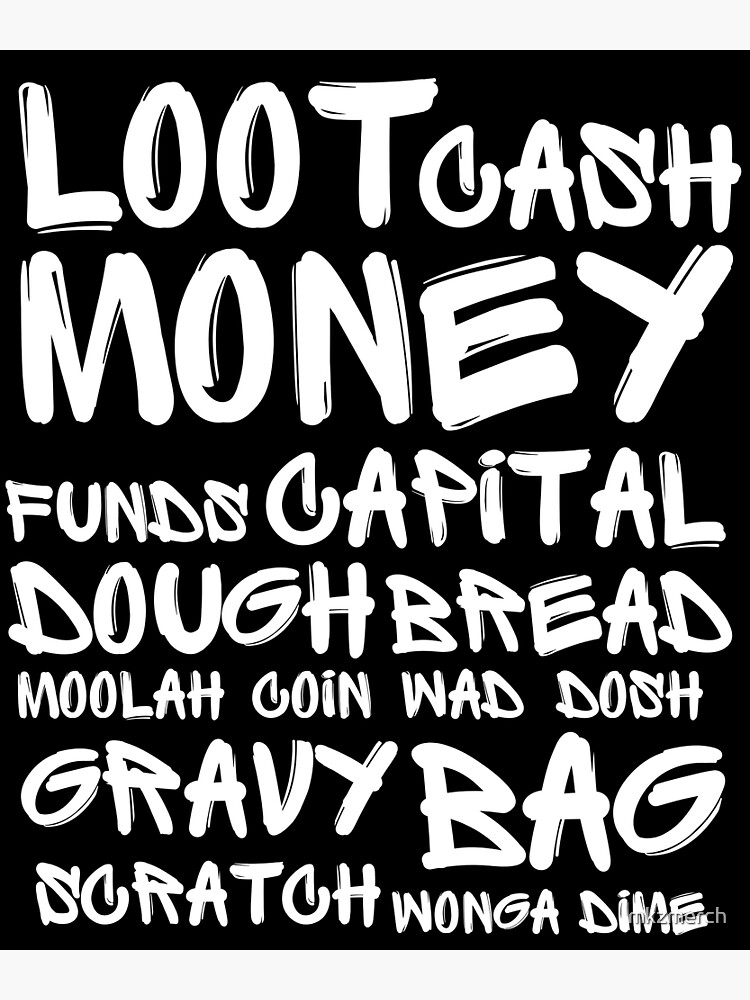This is a detailed black and white poster with a stark black background and bold white text, designed to resemble hand-painted strokes. The text appears in a stylized font that evokes the look of paintbrush lettering, complete with uneven areas where the black background peeks through, adding to the artistic feel. The poster prominently displays a series of slang terms for money, each listed on separate lines. From top to bottom, it reads: "loot, cash, money," followed by "funds, capital," then "dough, bread," "moolah, coin, wad," "dosh, gravy, bag," and finally "scratch, wonga, dime." At the bottom right corner, there is small text that reads "MKZ Merch," suggesting a branding element, possibly indicating it's part of a merchandise line. Overall, the poster emphasizes the diverse slang used for money, presented in a visually striking way.